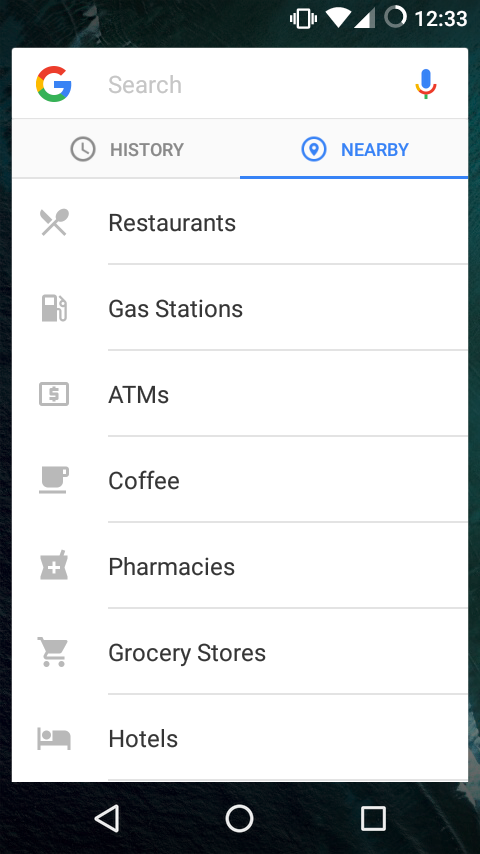This image is a close-up screenshot of a cell phone displaying the Google search interface. In the upper right-hand corner, there are the standard cell phone icons indicating battery life, signal strength, and Wi-Fi connection. Below these icons, the Google search bar sits prominently, although it is partially cut off on the left and right sides. The search bar itself is empty, and beneath it are two tabs: 'History' and 'Nearby'. The 'History' tab, accompanied by a clock icon, is grayed out, while the 'Nearby' tab is highlighted in blue with a blue underline, signifying it has been selected.

Below these tabs, a series of seven rows display various icons and corresponding labels for different locations: "restaurants," "gas stations," "ATMs," "coffee," "pharmacy," "grocery stores," and "hotels." Each row consists of an icon to the left of the label, making it easy to identify the type of location at a glance. This organized layout helps users quickly access nearby amenities based on their needs. The current time displayed in the upper right corner is 12:33.